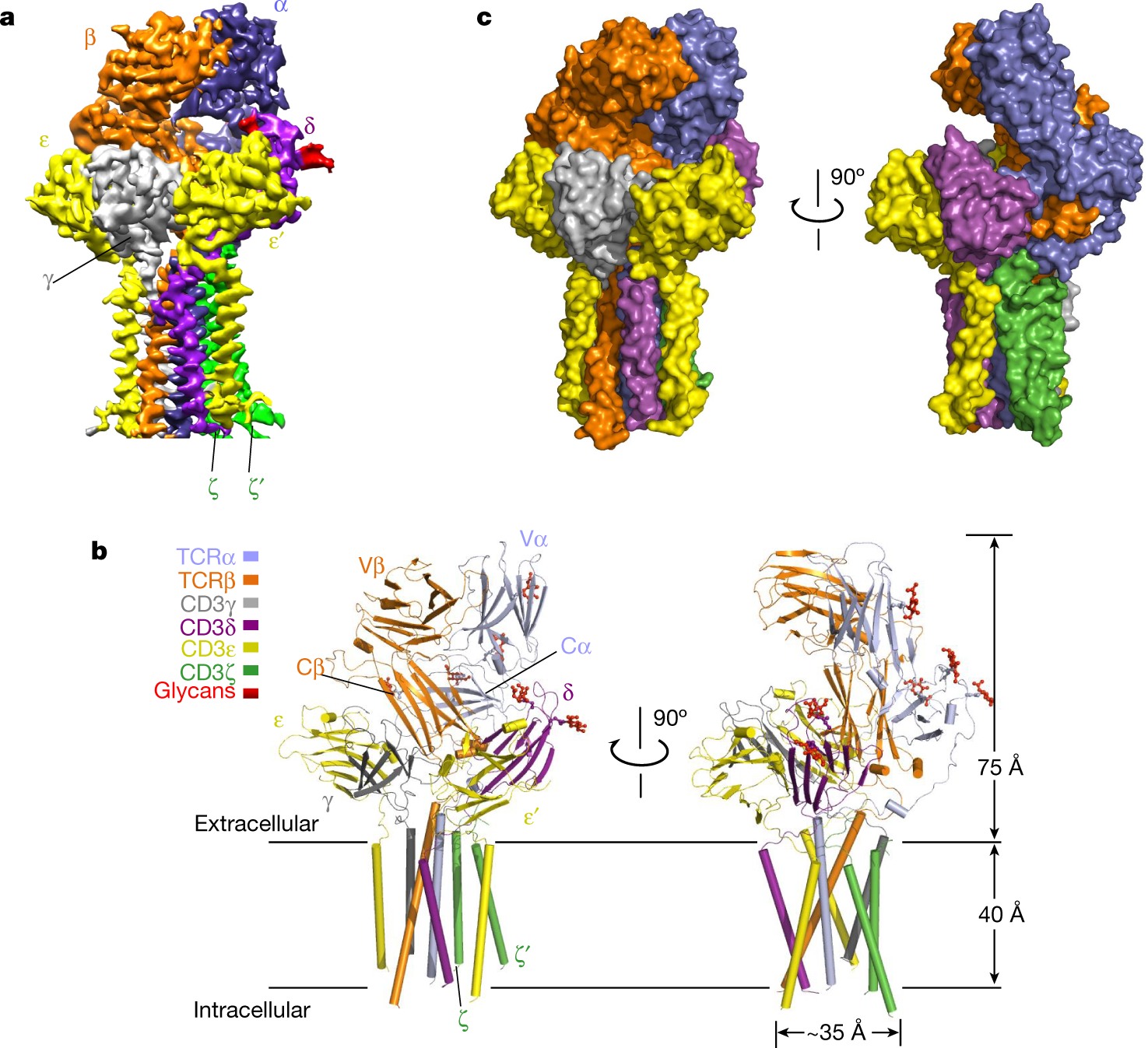The image is an intricate color illustration infographic in a landscape orientation, depicting various views of cellular structures. Dominating the upper half of the image, three distinct cellular structures are arranged side-by-side. The illustration on the top left, labeled 'A,' features a tree-like form with a large trunk and colorful clusters in shades of orange, blue, yellow, green, and purple. Adjacent to it on the right, another similar structure is labeled 'C,' shown twice, with one appearance rotated by 90 degrees. Below 'C,' a third structure is marked with the letter 'B,' accompanied by a color guide detailing scientific notations.

In the bottom section of the image, two blowout diagrams provide an enlarged view of portions of the cellular structures, highlighting specific parts with meticulous labels. Notably, the image identifies different regions with text labels and corresponding colors: orange for beta, purple for alpha, yellow for epsilon, pink for delta, white for gamma, and green for epsilon prime.

The labels 'extracellular' and 'intracellular' are located at the lower left corner, emphasized by black text. Beside these, elongated, pencil-shaped rods in colors yellow, orange, blue, light blue, green, and purple stretch upwards, forming streaks. Additionally, clusters of spirals in varying colors like yellow, brown, purple, green, and blue expand at the top, giving them the appearance of tree tops. Despite their complex and decorative arrangement, the specific scientific identification of these illustrated structures remains intricate and layered, ultimately creating a visually compelling display of cellular illustrations.